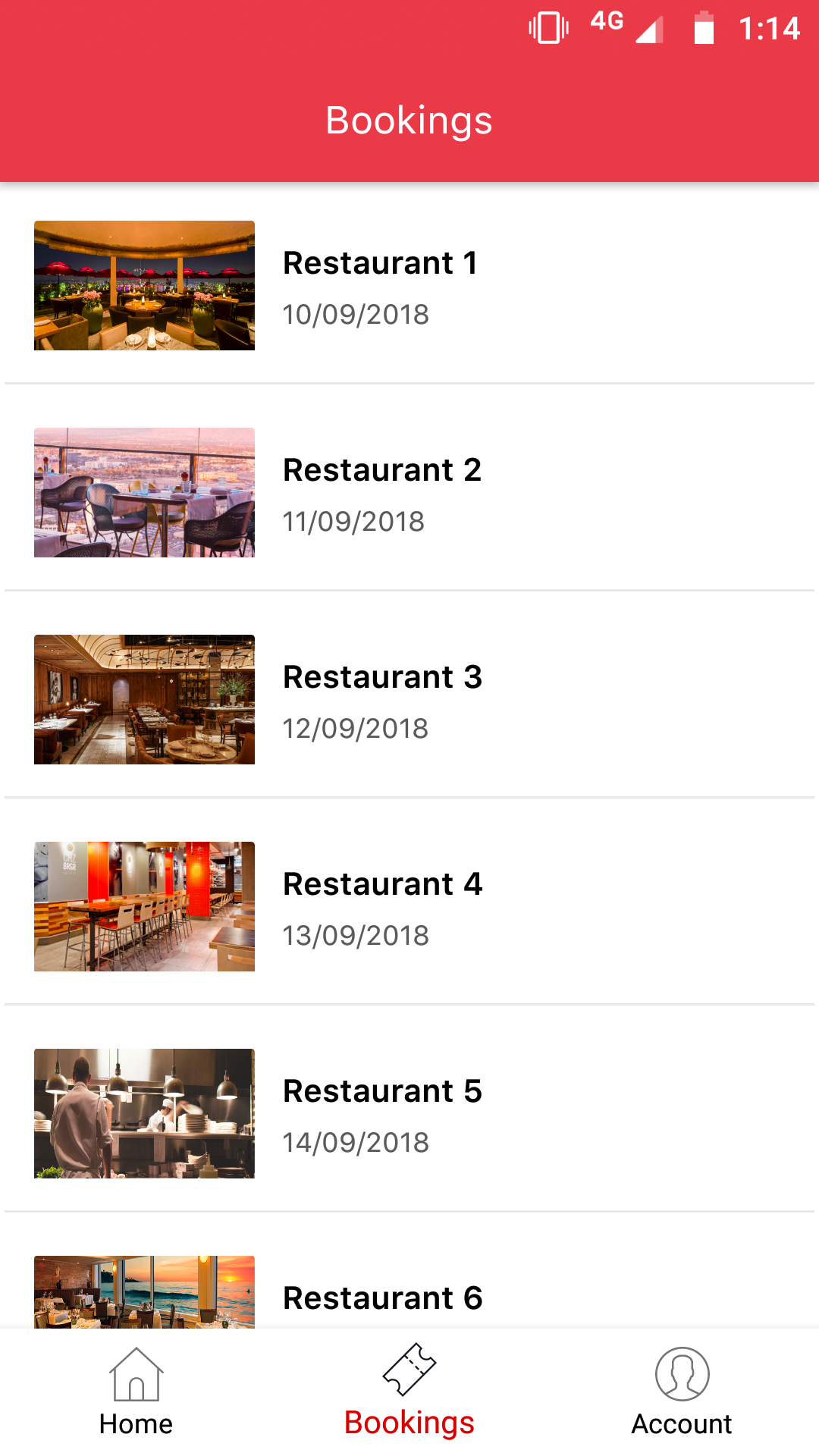This is a detailed screen capture from a smartphone displaying a list of potential restaurant bookings. The screen has a simple and straightforward design. At the top, against a red background, the header reads "Bookings." In the upper right corner, several status icons are visible, indicating the phone is on vibrate mode, connected to a 4G network, and showing the volume and battery levels. The time displayed is 1:14.

Beneath the header, there is a list of six restaurants, each labeled sequentially from "restaurant 1" to "restaurant 6." The listings include corresponding dates, starting from 10.09.2018 for "restaurant 1" and following a consecutive day-by-day pattern down to 14.09.2018 for "restaurant 5." The date for "restaurant 6" is partially cut off, but it logically follows that it would be 15.09.2018. Adjacent to each restaurant listing, there is an image showcasing the restaurant's interior, suggesting that they are all upscale establishments, including Asian fusion, balcony-type, and sushi restaurants.

At the bottom of the screen, three icons are displayed: "Home," "Bookings" (which is currently highlighted), and "Account."